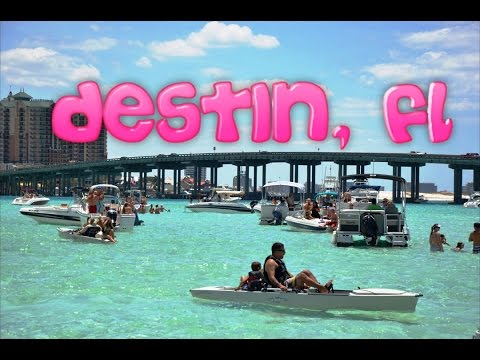In the photo, a variety of boats, both large and small, are scattered across the blue-green, shallow waters. People can be seen swimming and enjoying their time on paddle boats and small party boats. The setting is clearly in a tropical area with warm weather. In the distance, a large bridge spans the water, accompanied by what appear to be condominiums or a hotel on the left side. The sky above is a perfect blue adorned with white clouds. The text "Destin, Florida" is prominently displayed in pink. The scene is vibrant, featuring colors like blue, white, brown, tan, pink, gray, green, and red. The arrangement of the boats and people is random, giving a lively and bustling atmosphere.